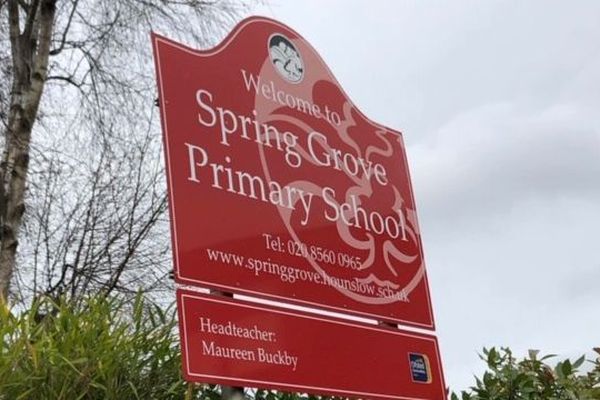This color photograph, taken on a cloudy day, captures an outdoor setting with a detailed shot of a red metal sideboard sign standing amid green grass and sparse vegetation. Dominating the center of the image, the sign reads, "Welcome to Spring Grove Primary School," in white outlined letters with a dome-shaped top. Below this welcoming message, the contact details are provided: "Telephone: 020-8560-0965" and the website "www.springgrove.hounslow.sch.uk." A smaller attached sign beneath the main board bears the name, "Headteacher Maureen Buckby." Positioned against the backdrop of a gray, overcast sky, the sign is held by two metal posts, flanked on the left by a tree with bare branches and interspersed greenery. The clarity of the photograph emphasizes the stark contrast between the bright red sign and its surrounding muted natural elements.